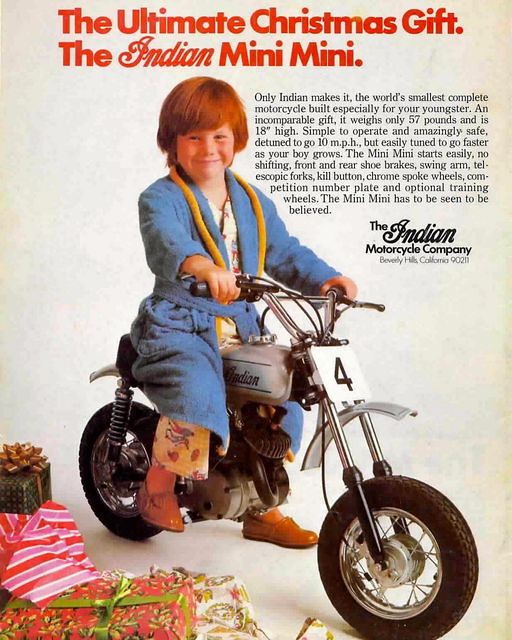The advertisement appears to be from the 1970s, featuring a faded photograph that reflects the era through the clothing and colors. The primary image shows a young boy, likely around four years old, with shaggy red hair, smiling and clad in a light blue bathrobe and pajamas. Interestingly, he’s also wearing shiny brown shoes, an odd combination with his sleepwear. The boy is sitting on a silver mini motorcycle labeled "Indian," reminiscent of a classic Indian motorcycle but scaled down for children. The backdrop is completely white, emphasizing the boy and the motorcycle.

Above the photograph, bold red text proudly proclaims, “The Ultimate Christmas Gift: The Indian Mini-Mini.” Beneath it, in smaller black font, a detailed description reads: “Only Indian makes it. The world’s smallest complete motorcycle, built especially for your youngster. An incomparable gift, it weighs only 57 pounds and is 18 inches high. Simple to operate and amazingly safe, detuned to go 10 miles per hour, but easily tuned to go faster as your boy grows. The Mini-Mini starts easily, no shifting, front and rear shoe brakes, swing arm, telescopic forks, kill button, chrome spoke wheels, competition number plate, and optional training wheels. The Mini-Mini has to be seen to be believed.”

Offsets towards the middle-right of the page, the company details are listed: “The Indian Motorcycle Company, Beverly Hills, California, 90211.” To the lower left of the boy, a pile of Christmas presents, both wrapped and unwrapped, further setting the festive scene, suggesting that it's Christmas morning and the boy is delighted with his new gift.